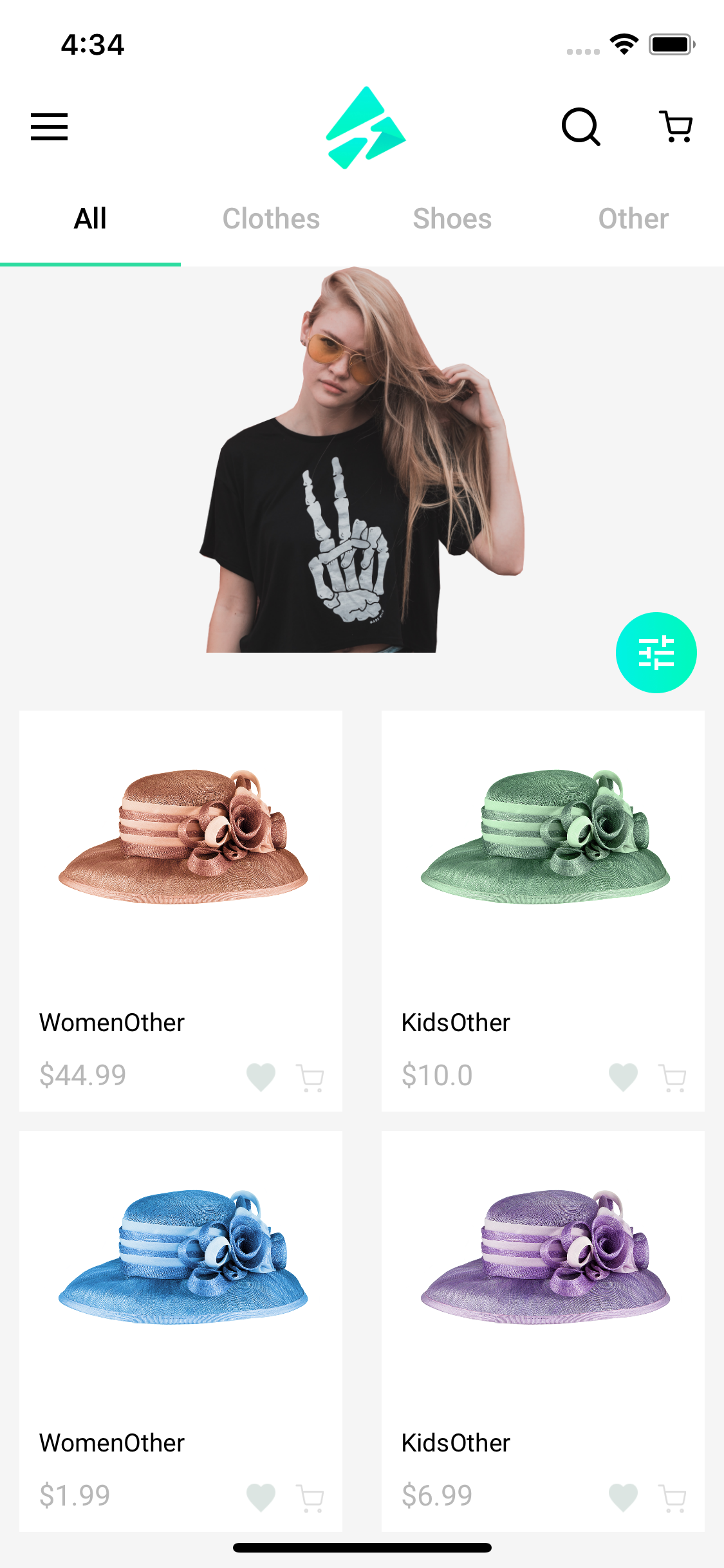The screenshot depicts a comprehensive interface of a shopping website.

At the very top, in black font, the current time is displayed as 4:34. Adjacent to the time on the right side, there's an icon for the Wi-Fi signal followed by a battery indicator. Below this, three horizontal lines are stacked, presumably representing a menu icon.

Centrally positioned is the shopping store's logo, colored in turquoise. Flanking the logo are a black magnifying glass icon symbolizing search functionality and a black shopping cart icon.

The navigation bar follows, featuring the categories "All," "Clothes," "Shoes," and "Other." The "All" category is highlighted in darker text, and beneath this bar is an accentuating green line. The rest of the interface has a light gray background.

Highlighted centrally is an image of a girl on this light gray background. She sports a black, short-sleeved t-shirt. The t-shirt boasts a graphic featuring a skeletal hand making a peace sign. She is adorned with sunglasses, and her blonde hair elegantly drapes over her left shoulder.

Below the image, there are four square sections each displaying different hats. 

The first square, colored peach-brown, reads "Women, Other, $44.99."
The next square is sage green and indicates "Kids, Other, $10."
Under the peach-brown square, a blue one is present with the text "Women, Other, $1.99."
The last square, in purple, states "Kids, Other, $6.99."

Each square succinctly labels the category, target demographic, and price of the item.